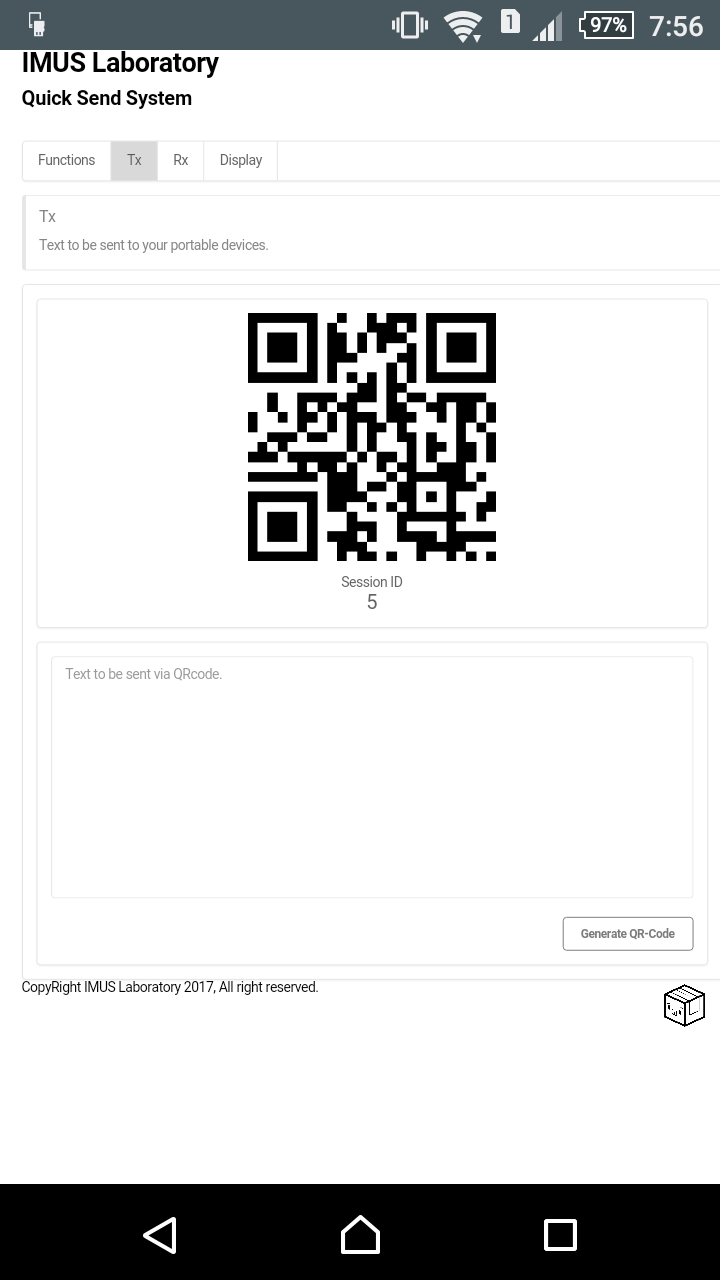This image is a screenshot of an outdated mobile device screen. The upper portion of the screen displays typical status indicators including the clock, battery life, and signal bars, all with an antiquated design. The main interface showcases an application titled "IMUS Laboratory," with a subtitle "QuickSend System." Following this, there are sections labeled "Functions," featuring "TX," "RX," and "Display." Beneath these, it reads "TX, text to be sent to your portable device." Centrally placed is a large QR code, accompanied by a session ID number 5. Below the QR code, the text indicates "Text to be sent via QR code." Adjacent to this is a button labeled "Generate QR code." At the bottom of the screen, the copyright notice reads "IMUS Laboratory 2017 All Rights Reserved." The interface predominately uses a white background with black text, organizing information into distinct boxes. The upper part of the device's exterior is dark grey while the lower part is black, featuring navigation icons for back, home, and multitask. The overall design of the application is minimalistic and somewhat visually unappealing. The purpose of the IMUS Laboratory system is not clear, though it possibly relates to medical testing or data transmission, as inferred from the context and terminology like "TX" suggesting transmission.